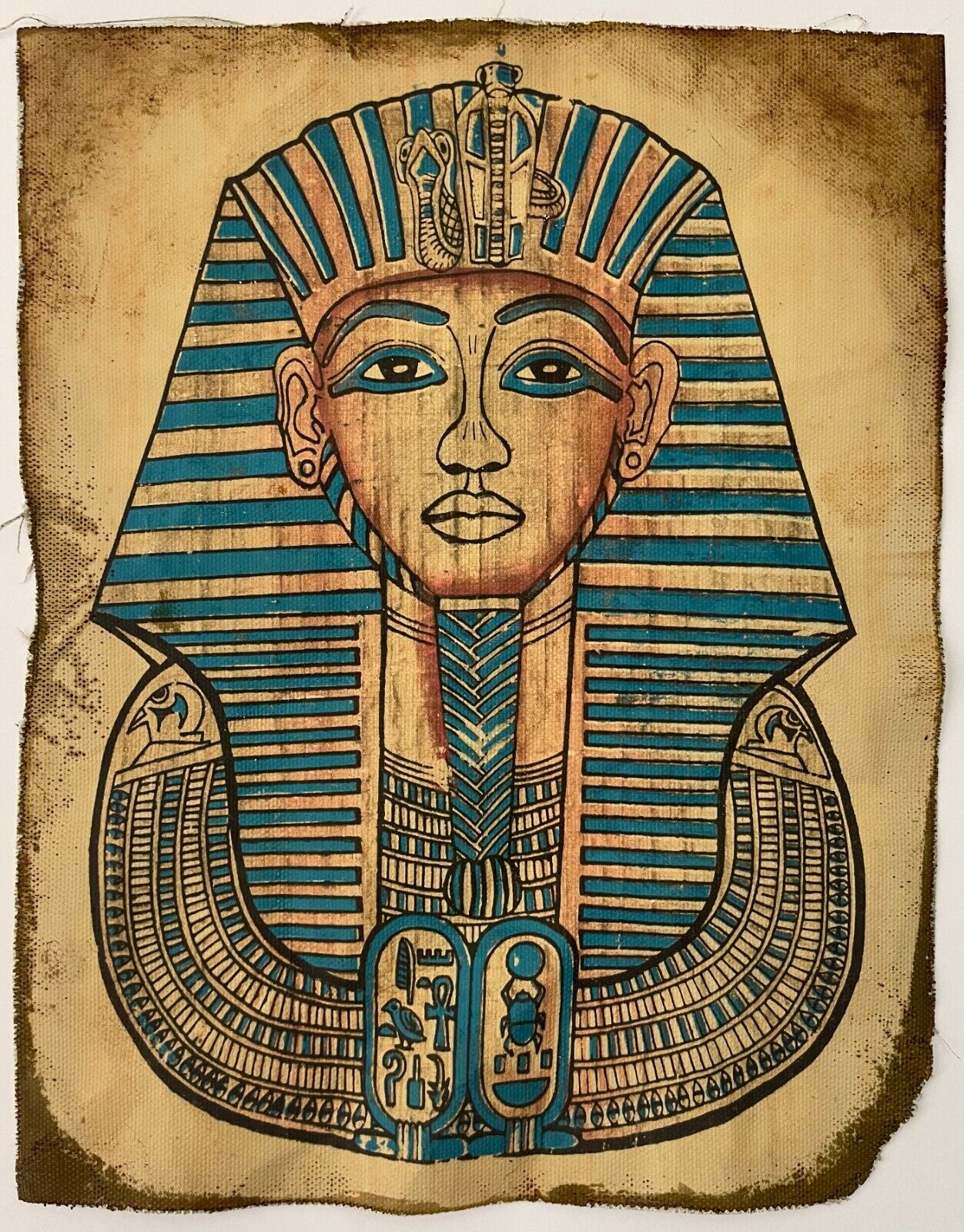The image depicts an illustration on an old, worn fabric that resembles parchment or burlap, with dark brown, frayed edges and a notably rounded, torn bottom right corner. Central to the illustration is a detailed, somewhat cartoony representation of King Tutankhamun's golden funerary mask. The pharaoh's face, depicted in a gold-tan color, is adorned with a distinctive Egyptian headdress that extends well below the shoulders, featuring horizontal and vertical blue stripes and two cobras at the crest. The pharaoh's facial details include blue eyebrows, blue winged eye makeup, and a long, braided blue goatee. Below the depiction of the head, there are hieroglyphics encased in oval cartouches upright, and a large, intricately designed necklace with medallions around the shoulders, detailed with blue squares, bird imagery, crosses, and a scarab beetle.